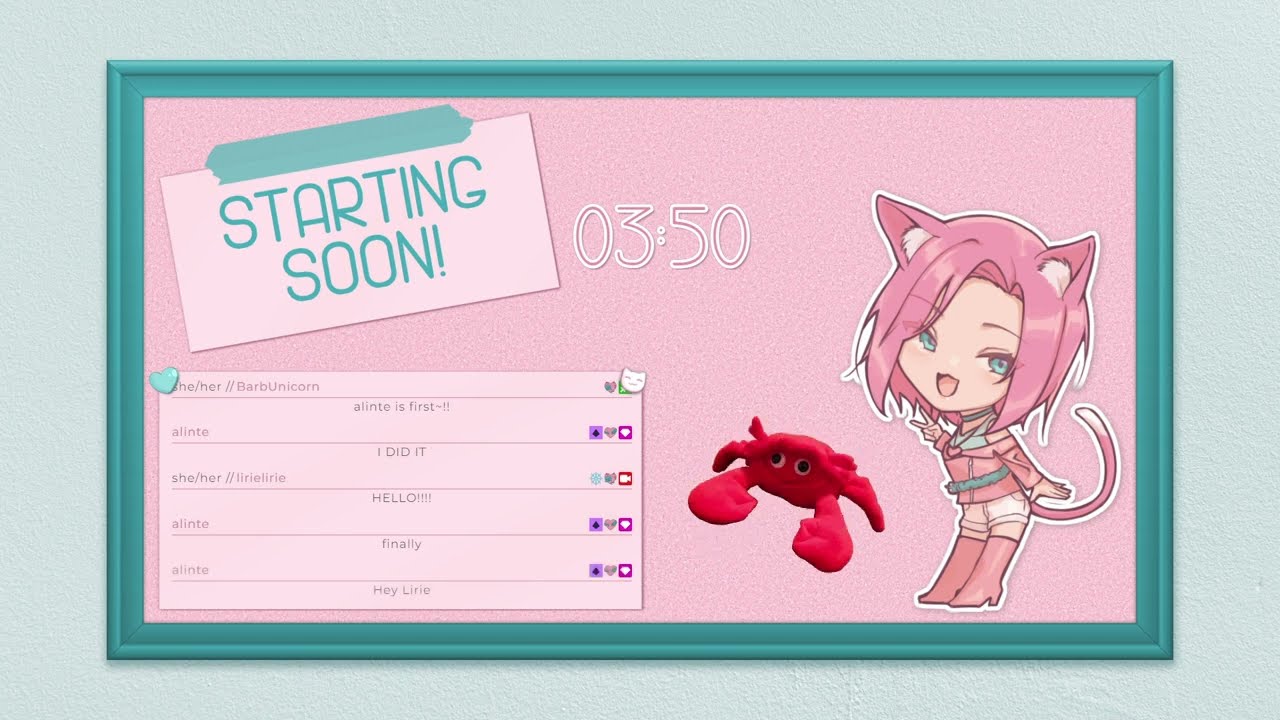The image features a wide rectangular sign with a light blue background, framed by a teal blue wooden border. Inside, there is a prominent pink board. In the upper left-hand corner of this pink board, there is a piece of aqua mint tape displaying the message "Starting Soon." Centered on the board is the time "03:50." Below the time, there is a section for writing with various messages such as "I did it," "hello," "finally," and "hey." 

On the right-hand side of the board, there is an anime-style female character with pale skin, blue eyes, and vibrant pink hair. She has pink cat ears, a pink cat tail, and is dressed in a pink outfit with a teal belt. Next to her, closer to the center, is a small red crab. The left side of the board contains a list, including phrases like "she," "her," and other small text resembling a social media profile.